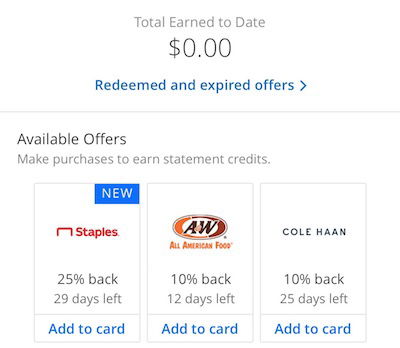The image is a screenshot of an online offers page, prominently displayed against a white background. At the top center, written in gray font, is the text "Total Earned to Date," followed by "$0.00" in bold black and gray letters. Below this, in blue font, is a clickable link labeled "Redeemed and Expired Offers," accompanied by a right-pointing arrow, suggesting it opens more options when clicked.

The page is bordered by a thin black line, and below the link, a light gray subheader reads, "Available Offers. Make purchases to earn statement credits." Three offer boxes are neatly arranged under this subheader, showcasing different promotions.

The first box features an offer from Staples, highlighted by a blue "New" button in the top right corner. It promises 25% back with 29 days remaining and an "Add to Cart" option in blue font. The Staples logo is positioned to the left.

The middle box presents an offer from A&W All American Food, offering 10% back with 12 days left, and similarly includes an "Add to Cart" button.

The third box on the right is for Cole Haan, offering 10% back with 25 days remaining, also featuring an "Add to Cart" button.

Each offer is visually consistent, maintaining the white background and gray font, creating a clean and organized layout for the user to interact with.